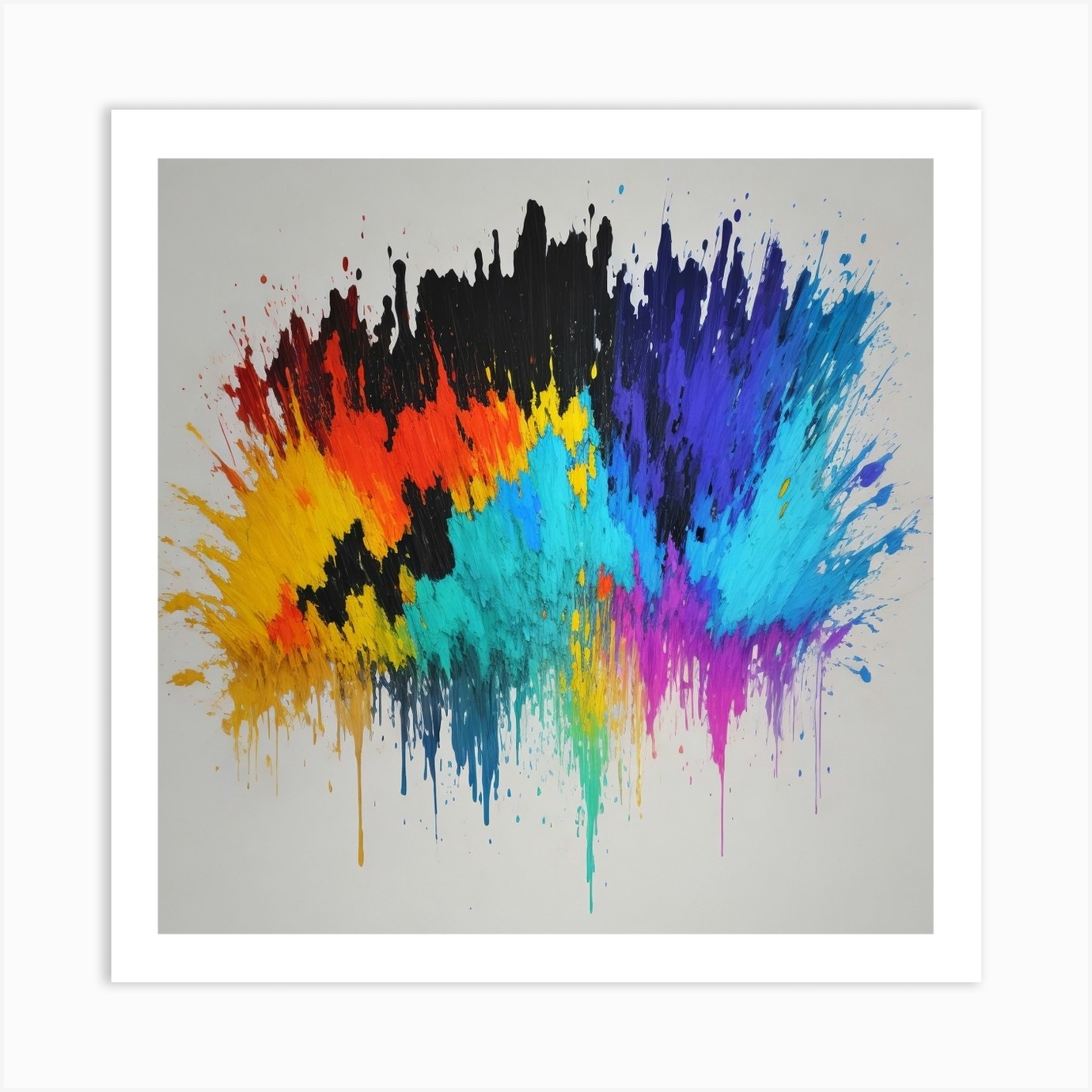This captivating image features a digital recreation of an abstract painting with a striking array of vibrant colors, including splashes of yellow, orange, black, teal, light blue, dark blue, dark purple, magenta, and pink. The colors appear to be whimsically thrown and allowed to drip and blend into each other, creating an energetic and dynamic composition. Set against a dark gray background, the artwork is framed by a crisp white border that gives it the polished look of a photograph, reminiscent of a Polaroid's signature style. This colorful, nearly rainbow-like piece stands out vividly and seems as if it could be displayed in an art gallery, celebrated for its free-spirited and expressive nature. The overall presentation is completed with a drop shadow, enhancing its depth and making it visually striking against a plain white backdrop.